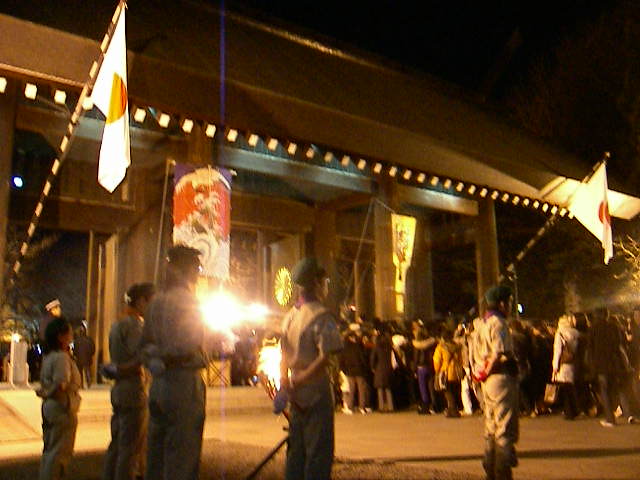This photograph captures a nighttime procession in front of an Asian, likely Japanese, temple. The scene is illuminated by bright lights coming from the building’s entrance, casting a glow on the numerous people gathered. A group of approximately five individuals, dressed in khaki uniforms with red sashes and green berets, stand with their right arms behind their backs and their left arms down. They appear to be part of a formal ceremony, possibly a military or scout event, given their uniforms and disciplined posture.

Two Japanese flags, white with red circles, are prominently displayed and partially crinkled on their poles. These flags and additional indistinguishable banners are draped across the temple entrance. An audience is gathered beyond this group, composed of men and women, huddled around the building. The background also reveals a gate and additional structures, enhancing the temple's prominence in the image.